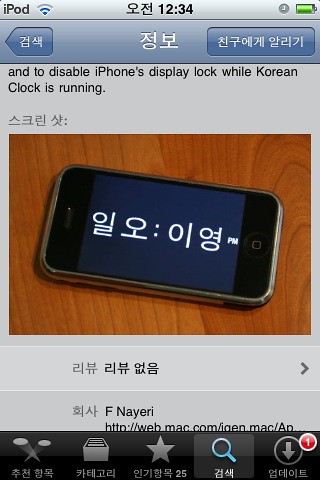This image displays a screenshot captured from an iPod, as indicated by the text at the top of the screen. The status bar reveals the Wi-Fi signal strength, the time set at 12:34, and the current battery level. The main content of the screenshot includes a message explaining how to disable the iPhone's display lock while a Korean clock app is running. Below this text, there is a photograph of an iPod placed on a wooden tabletop, featuring a Korean clock on its display. At the bottom of the screenshot, various icons are visible: a star, a magnifying glass, and an arrow pointing downwards encased in a circle. Additionally, there is some Korean text present on the screen.